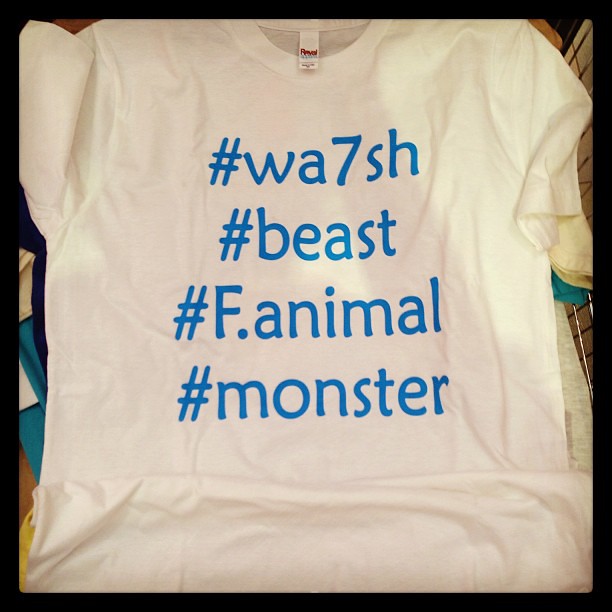This is a vertical rectangular color photograph of a white cotton, short sleeve crew neck t-shirt, prominently printed with bold text in the center. The text is composed in a bright turquoise blue and features a series of hashtags: "#WA7SH," "#beast," "#F.animal," and "#monster," arranged vertically. The photograph is bordered thickly in black, creating a framing effect. The shirt appears to be positioned on the top of a stack of other t-shirts, with the sleeves of adjacent t-shirts peeking through the edges—specifically, one in a light orange, another beige, and a third possibly in turquoise. There are hints of a metallic object on the right, which could be part of a shopping cart or fenced area, adding a hint of context to the setting. The background is cream-colored, providing contrast to the bright white shirt and its vivid print.